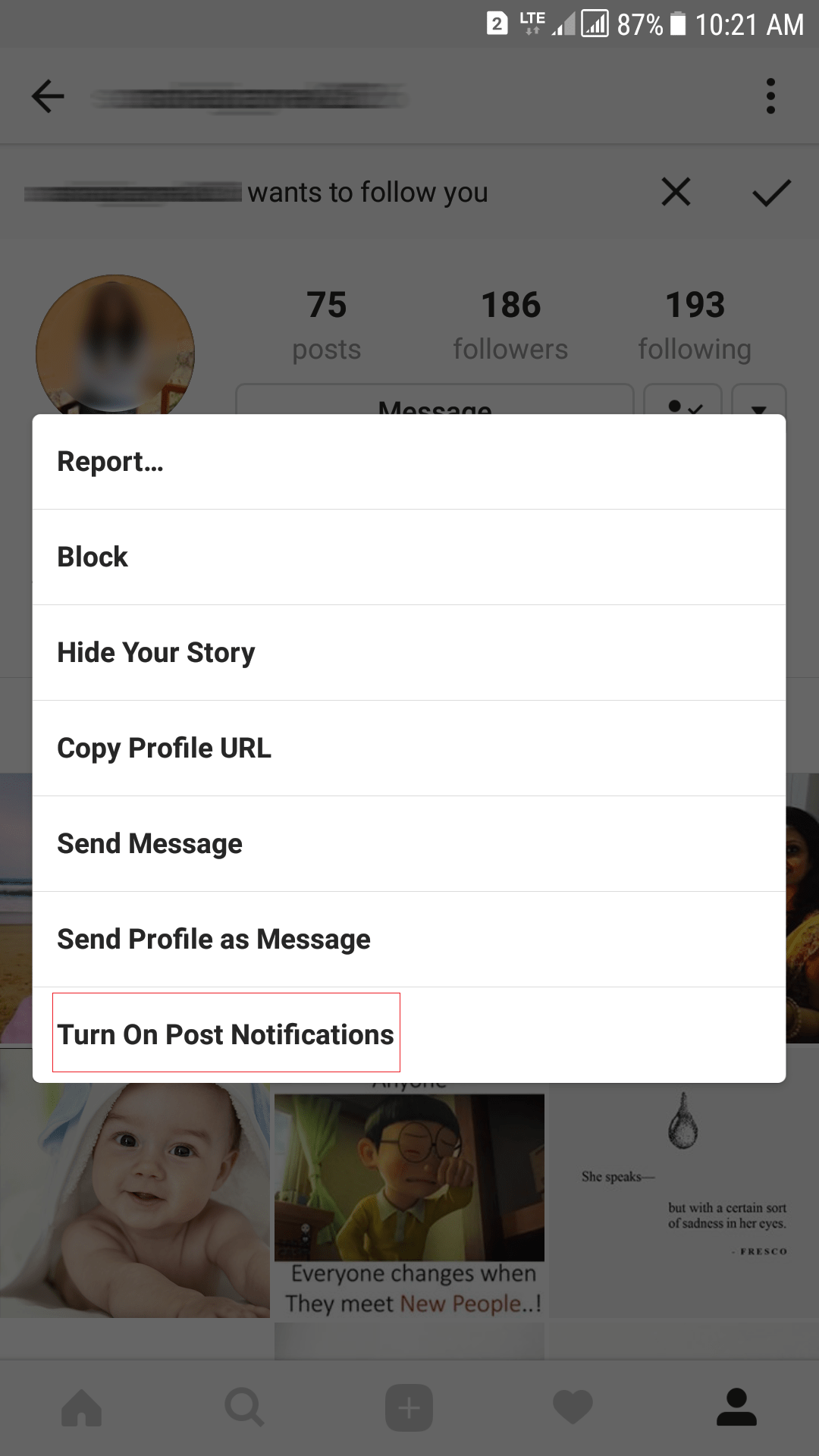The image is a detailed screenshot of a smartphone display. In the upper left-hand and right-hand corners of the screen, white text and icons are visible against a gray backdrop. On the right side, a blue page with a gray tube is shown, with the letters "LTE" next to it, indicating the network connection. Following that are the signal bars representing phone service strength and a white box with blue service bars indicating WiFi. Adjacent to these icons is "87%" showing the battery level, followed by a battery icon. The time displayed is "10:21 AM."

The background of the screen appears to be a Facebook or Instagram page, but it is slightly dulled with a gray haze. On the left side, there is a yellow circular icon featuring someone's profile picture. Overlaid on this backdrop is a white pop-up box with black text options listed vertically. The top option reads "Report" followed by three dots, below it is "Block," "Hide Your Story," "Copy Profile URL," "Send a Message," "Send Profile as Message," and "Turn on Post Notifications," which is circled by a thin red box.

Beneath the pop-up box, the underlying page shows part of an image, featuring what appears to be a Caucasian baby partially wrapped in a blanket that drapes around its head. Next to the baby is a CGI-style cartoon character of Asian descent, dressed in a yellow shirt with a white collar and round glasses. The character is depicted crying and raising a hand to wipe away tears.